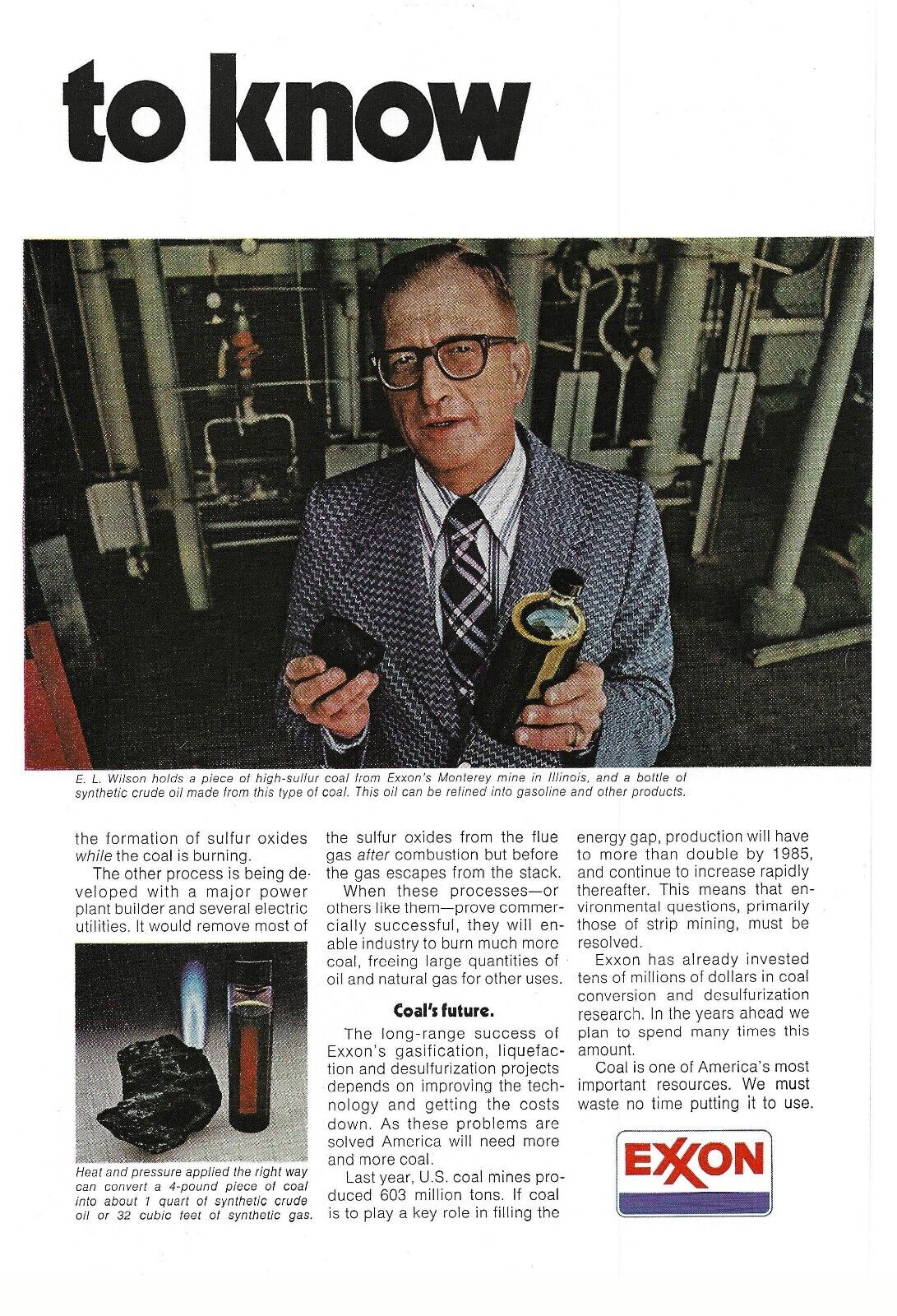The image appears to be a scanned newspaper or magazine article titled "To Know," featuring a detailed discussion about Exxon’s coal gasification process. At the top of the article, the headline "To Know" is written in lowercase black text. The main photograph showcases an older man with short hair parted on the left side, wearing glasses, a black and white checkered suit, and a black and white lined tie. He is identified in the caption as E.L. Wilson. In the image, Wilson is holding a piece of high sulfur coal from Exxon’s Monterey Mine in Illinois in his right hand and a bottle of synthetic crude oil made from this coal in his left hand. The caption explains that this synthetic crude oil can be refined into gasoline and other products. In the background, there appears to be complex machinery, giving the impression of an industrial setting. Below this main image, there is additional text and another smaller photograph depicting a piece of coal and a vial with a dark liquid, presumably synthetic crude oil. The bottom right corner of the article features the Exxon logo in red text with a dark blue line underneath it. Overall, the article discusses the long-range success and the industrial process of converting coal into synthetic crude oil.